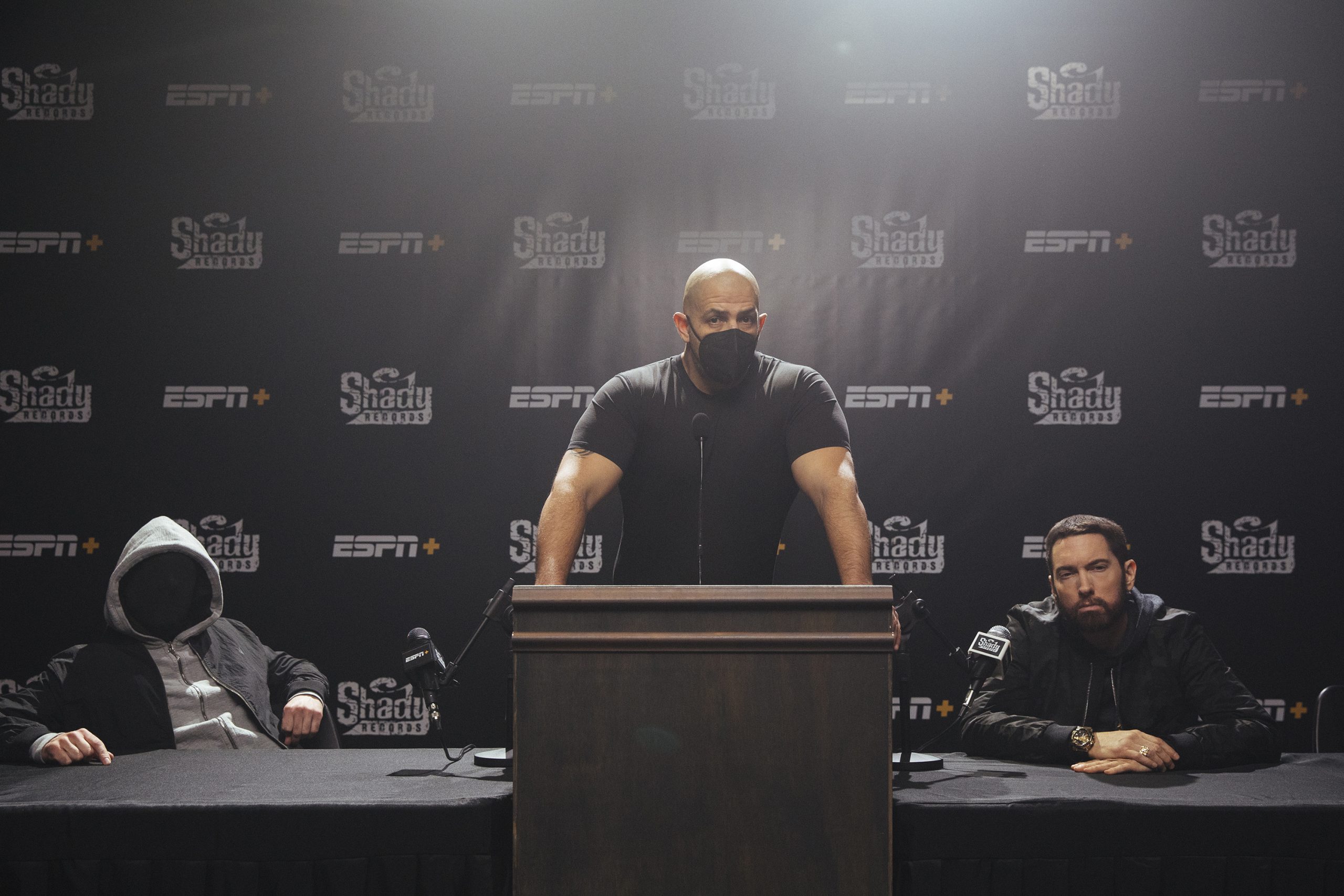In this image, a large, muscular man stands at a wooden podium, flanked by two serious-looking individuals at tables with black coverings. The man at the podium, wearing a black t-shirt and a COVID-type black face mask, has his hands braced on the podium, emphasizing his muscular arms. He has closely shaved hair and stands under a spotlight that highlights his tough appearance. Behind him, the wall is covered with alternating printed words "Shady Records" and "ESPN" in rows. On the right side of the image, Eminem sits at a table, wearing a black jacket. On the left side, another person, whose face is completely obscured by shadows and a hoodie, has visible white hands suggesting he is Caucasian and wears a dark jacket over the hoodie. The event appears to be related to both ESPN and Shady Records.